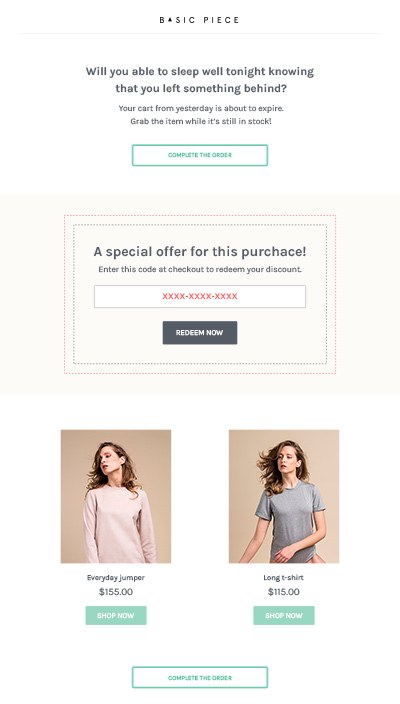On a white background, the image features a prominent purple-tinted box at the top with the heading "Basic Piece." Below the heading, text in purple reads, "Will you be able to sleep well tonight knowing that you left something behind? Your cart from yesterday is about to expire. Grab the item while it's still in stock." 

Beneath the message, a blue button with white text stands out, displaying "Complete the Purchase." Adjacent to it, a light purple box presents a special offer message: "Special offer for this purpose. Enter this code at checkout to redeem your discount."

Further down, there's a white box adorned with pink "X" patterns, followed by a sleek black box with white text that says, "Redeem Now."

At the bottom section of the image, two product snapshots are displayed featuring items and models:
- On the left, a model in a long-sleeve shirt priced at $155, accompanied by a blue "Shop Now" button.
- On the right, a model in a t-shirt priced at $115, also accompanied by a blue "Shop Now" button.

Lastly, another blue-buttoned "Complete the Purchase" prompt punctuates the bottom of the image, directing viewers to finish their transaction.